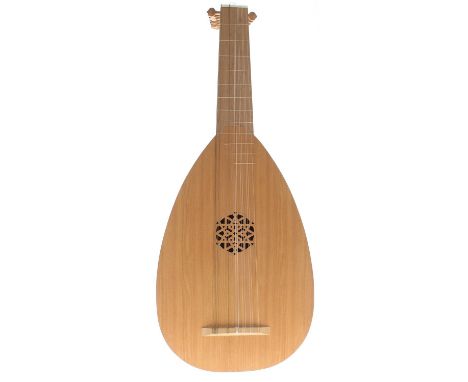The photograph features a striking string instrument with a rich medieval heritage, centrally positioned against a plain white backdrop. The instrument has a distinctive pear-shaped, oval, or oblong wooden body, which is predominantly a light wood color. The strings, likely made of a thin white material, stretch vertically from the bottom part of the instrument up towards the neck. At the bottom, there is a crucial connecting point for these strings.

In the middle of the body, there is an intricate, mandala or snowflake-like design around a circular sound hole, allowing the instrument's music to project. The neck, which extends out of the frame’s top, features horizontal lighter lines reminiscent of a guitar's frets, aiding in finger placement for playing. There are also protruding knobs at the top of the neck, presumably for tuning the instrument. With six pairs of strings, this mid-sized instrument looks like a forerunner of modern guitars or banjos, often depicted in medieval artwork.